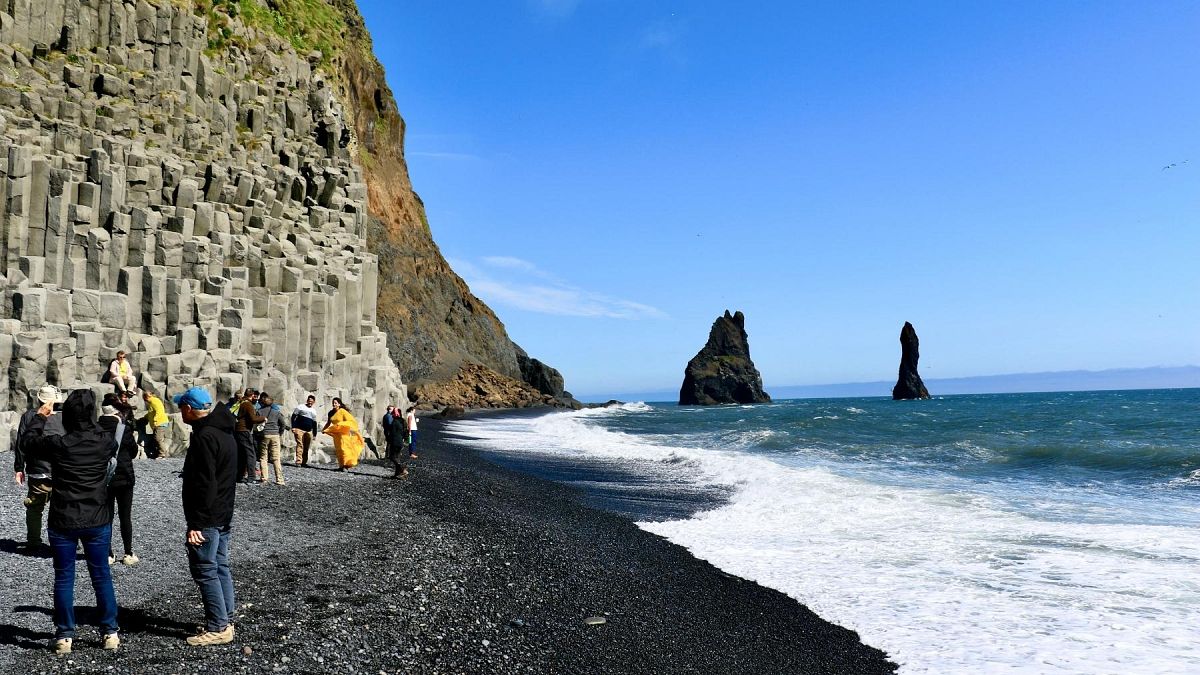The image depicts a striking beach scene where the dark green or dark blue ocean meets the shore, turning white as waves crash against it. The wet shore appears dark gray, gradually lightening to a pale gray towards the left-hand side of the image. Scattered across the shore are several people, many dressed in long-sleeved shirts and jeans. A standout figure is a woman in an all-yellow dress that billows in the wind, her dark hair contrasting against the backdrop as she walks towards the front of the image on the left side. Tall, gray rock pillars are stacked along the bank to the left, resembling a steep hill with rocks of varying sizes. The sky above is a clear, vivid blue, adding to the picturesque quality of the scene.